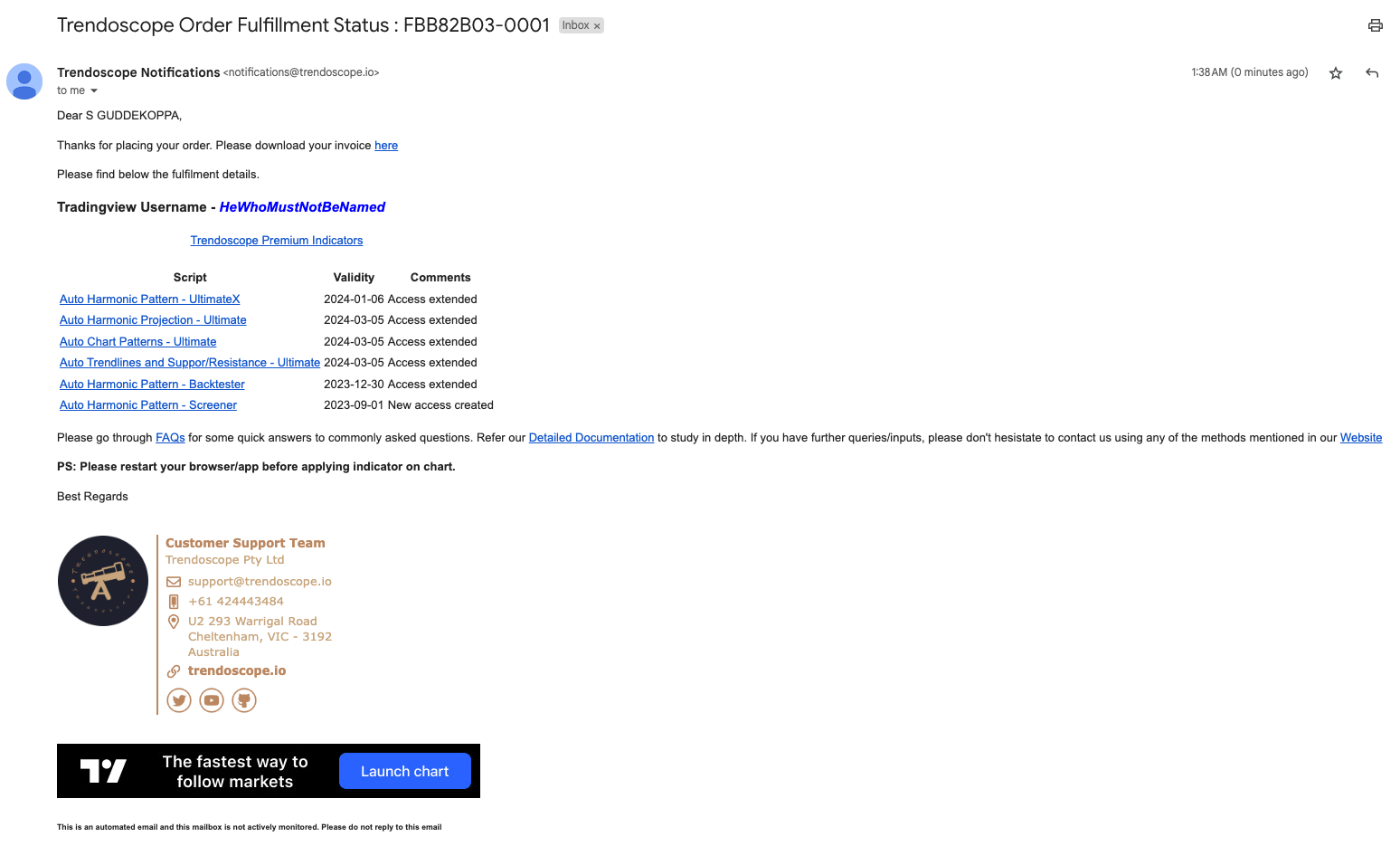**Detailed Caption:**

This screenshot showcases a webpage from the TrendScope Order Fulfillment Status section. The background is predominantly white with primarily black text and minimal use of color. 

At the top of the page, the heading reads "TrendScope Order Fulfillment Status" beside which an order number is displayed along with an inbox button to the right. Positioned on the left side is a blue icon featuring a darker blue human silhouette. Adjacent to this icon, the text "TrendScope Notifications" is written in dark black, below which an email address is provided.

The message starts with: "Dear S. Gudacopa, Thank you for placing your order. Please download your invoice [here]," with "here" being a clickable blue hyperlink. The message continues, detailing the fulfillment information with "Trading View Username" followed by "He Who Must Not Be Named" in bold blue fonts. Below this is another hyperlink, "TrendScope Premium Indicators."

The left-hand side of the page contains a three-column table with headers in black text: "Script," "Validity," and "Comments." Underneath the "Script" column, several hyperlinked product names are listed:
- Auto Harmonic Pattern Ultimate X
- Auto Harmonic Projection Ultimate
- Auto Chart Patterns Ultimate
- Auto Trend Lines and Support Resistance Ultimate
- Auto Harmonic Pattern Back Tester
- Auto Harmonic Pattern Screener

Opposite these product names under the "Validity" column, specific dates are mentioned with "Access Extended" noted to the right of each date.

Following the table, instructions are given: "Please restart your browser or app before applying the indicator on the chart." The message then closes with "Best Regards."

At the bottom, there is a large circular dark logo featuring a telescope on a stand pointing right. Adjoining the logo, in gold lettering, it states "Customer Support Team, TrendScope Pty Ltd." This section also provides an email address, phone number, and an address located in Australia, along with the URL "trendscope.io." Below this are three icons: Twitter, YouTube, and one that resembles a cat.

Finally, at the very bottom sits a black bar with white text stating "17, the fastest way to follow markets." To the right, there's a blue button labeled "Launch Chart."